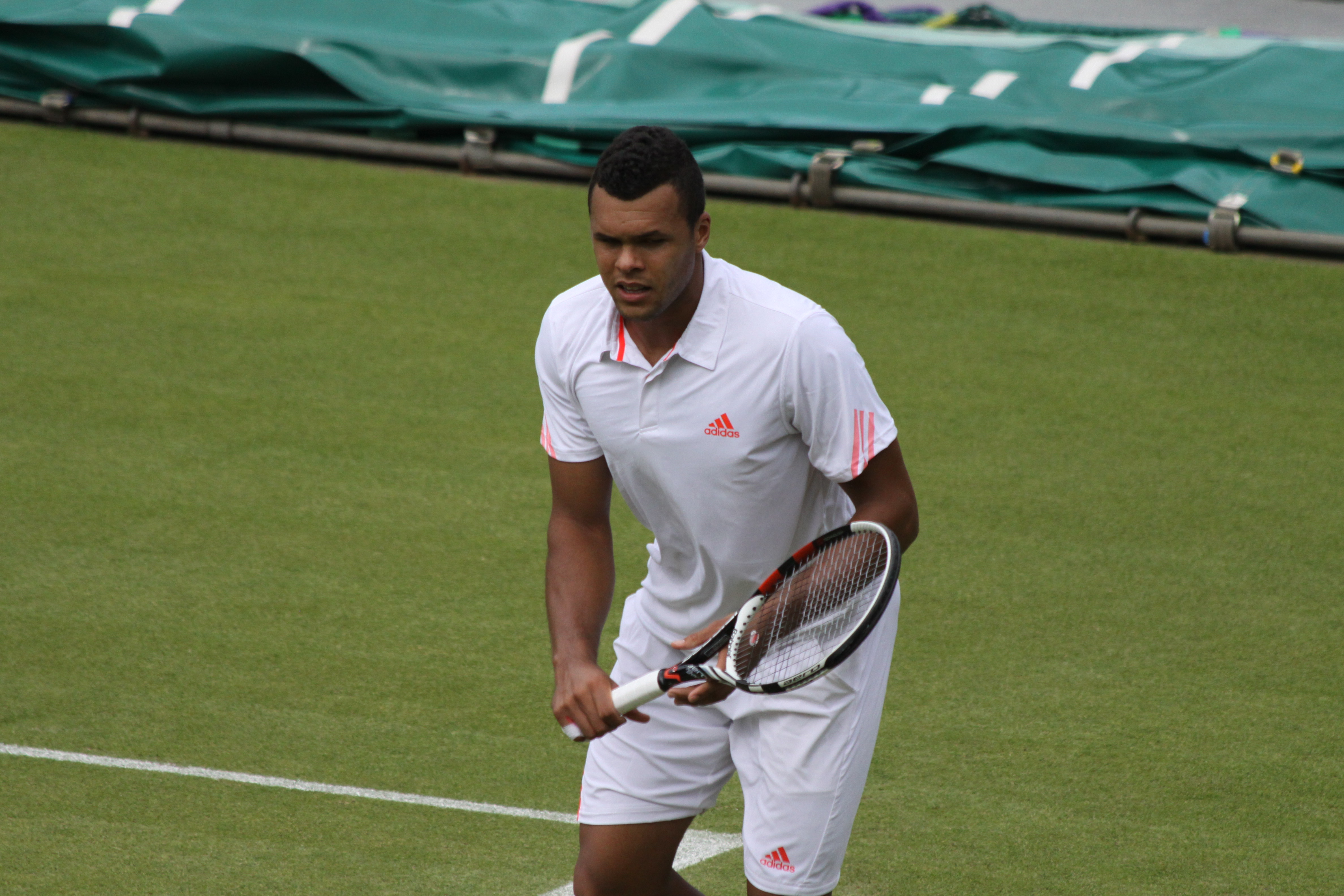In this detailed image, a young, dark-skinned Hispanic man stands confidently on a flat, green, grassy tennis court marked with white lines. Positioned centrally, he wears a white Adidas polo shirt accented with orange and matching white shorts, both displaying the Adidas logo. He grips a white tennis racket in his right hand while his left hand rests on his knee, as he crouches slightly with bent elbows and knees, looking straight ahead. His defined hairline and snow-white hair add a distinct contrast to his overall appearance. A green tarp with a black bar in the background suggests a protective measure against rain, highlighting the outdoor setting on what appears to be a clear day in the middle of the afternoon.